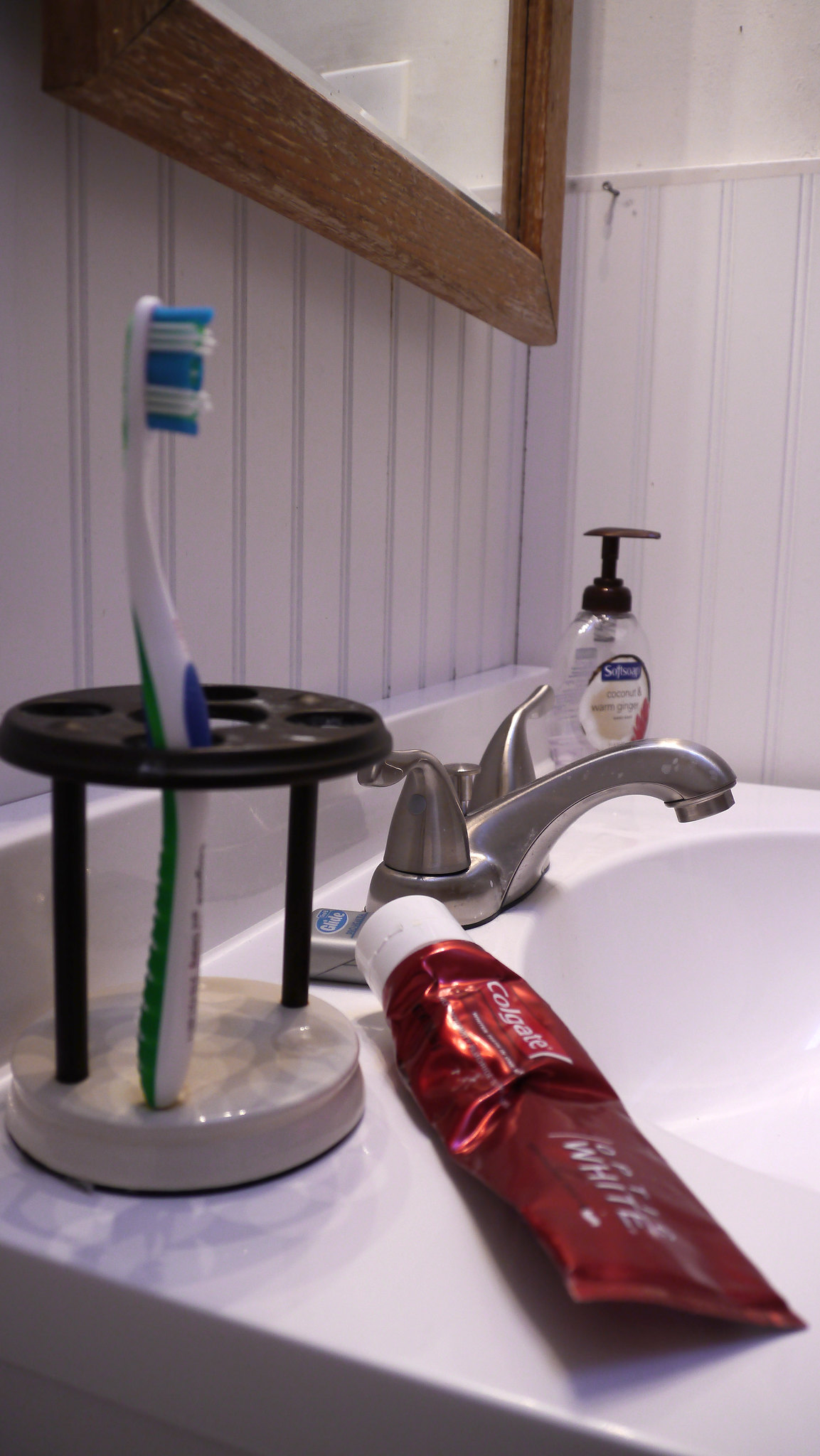In this close-up photograph of a bathroom sink, the scene captures a detailed view of the right corner of the room. The sink itself is a standard white porcelain basin, set against a limited counter space viewed from a low angle, almost level with the counter. Prominently displayed on the countertop is a red tube of Colgate toothpaste, possibly labeled with "whitening" text. Beside the toothpaste stands a toothbrush holder with a round marble base and a wooden support structure. The holder features four small slots, of which one is occupied by a toothbrush, and a central round slot likely intended for the toothpaste. Adjacent to the holder sits a compact container of Glide dental floss.

Next to the dental floss is the faucet fixture, a single unit equipped with two separate handles. Beyond the faucet, a bottle of Softsoap hand soap is positioned within easy reach. The walls around the sink are paneled in white wood, contributing to a clean and minimalist aesthetic. On the left side of the composition, a mirror with a wooden frame hangs on the wall, while on the right wall, a protruding nail is visible against the white paneling.